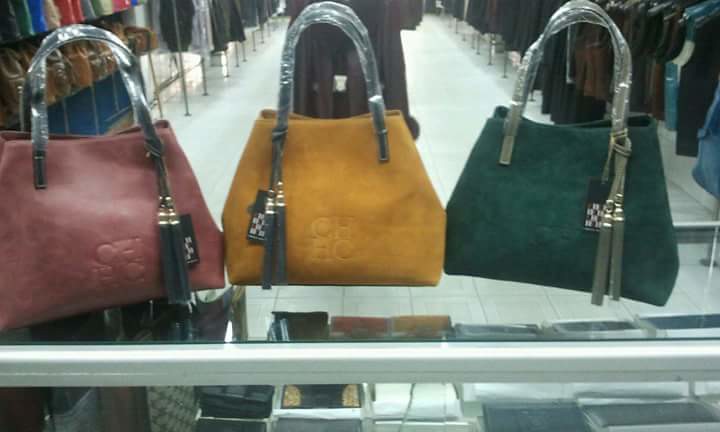This color photograph captures a display in a clothing store, showcasing three identically shaped trapezoidal handbags positioned atop a glass countertop. The countertop, edged with silver trim, reveals an assortment of women's leather wallets in various shades below it. The handbags, from left to right, are colored a dull brick red, gold, and dark forest green. Each handbag is equipped with a U-shaped handle, wrapped in protective plastic and featuring a gray or black tassel. Behind these handbags, the backdrop consists of racks filled with jackets and clothing, emphasizing the retail environment. Although the photograph is slightly out-of-focus, the repeated elements of black-wrapped handles, identical handbag shapes, and the presence of additional accessories below the glass case are clearly discernible.